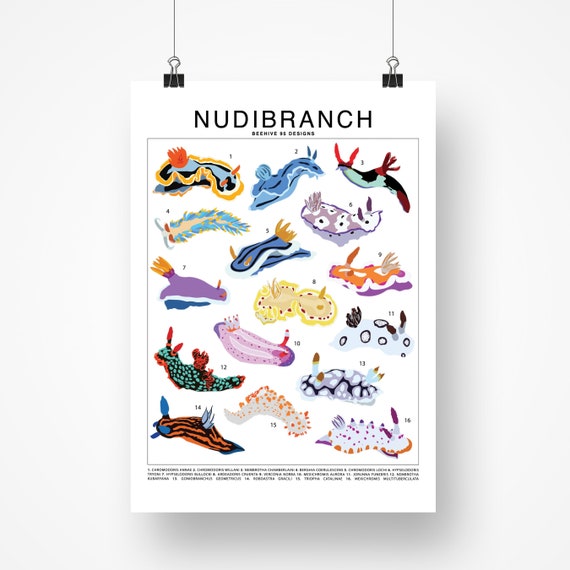The image is a vertically rectangular, full-color photograph showcasing a vibrant poster, held up by two black binder clips with silver handles, attached to pieces of string hanging from the top. The poster itself has a white background and is framed against a light gray, shadowed backdrop. At the top of the poster, the word "Nudibranch" is prominently printed in bold, capital black letters, with the text "N-U-D-I-B-R-A-N-C-H" underneath. Below the title, the poster features a collection of 16 detailed, artistic representations of nudibranchs, displayed in an array of vivid, unnatural colors including pinks, blues, and multicolored patterns. These illustrations vary in shapes and designs, resembling a mixture of slugs, sea anemones, and imaginary underwater creatures. Some figures are polka-dotted, some striped, and others have distinctive features such as small red antennae-like appendages. Despite the whimsical and varied appearances of the creatures, their exact nature remains ambiguous, adding to the intriguing and playful aesthetic of the poster.